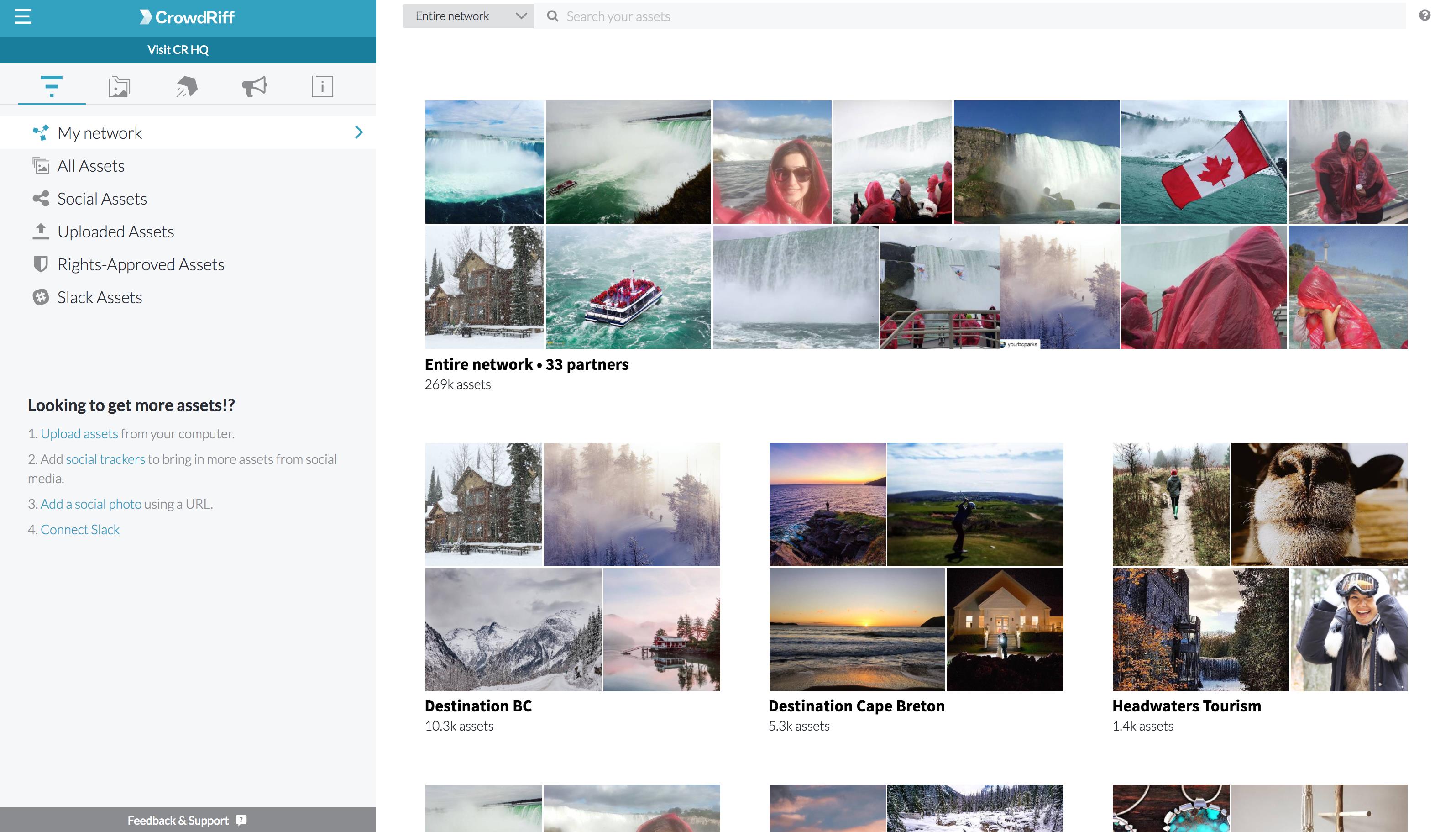The image displayed on the screen features an organized interface with various sections and labels. On the left side of the screen, multiple images are categorized and listed vertically. The top image is labeled "Entire Network, 33 Partners," signifying a collective group of associates. Below this are other categorized images labeled "Destination BC," "Destination Cape Britain," and "Headquarters Tourism."

Beneath these images, a blue label marked "Crowd RIF" is prominently displayed. Below this label, there is a set of listed options: "My Network," "All Assets," "Social Assets," "Uploaded Assets," "Right Approved Assets," and another option that appears to be "Sleek DAC assets." Each of these options likely serves as navigational links or categories for asset management within the network.

Further down the list, there is a prompt to "Get More Assets," suggesting additional resources or downloadable content, and at the bottom, a section labeled "Feedback and Support" is present, which is presumably a clickable link for users seeking assistance or wishing to provide feedback on the platform.